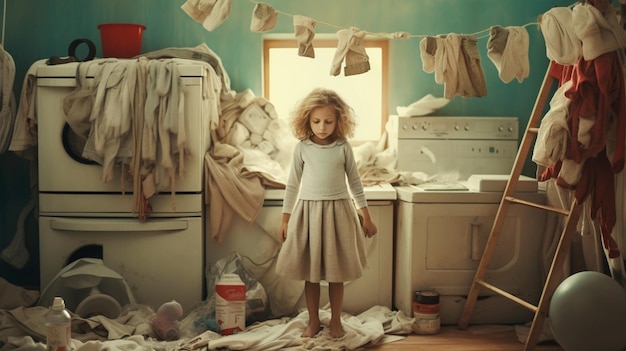In the center of a computer-generated depiction of a chaotic laundry room, a young, blonde-haired girl stands barefoot on a white cloth. She wears a white long-sleeve shirt with ruffles at the collar and a pink skirt. Her wavy hair extends to her shoulders, and her eyes are cast downward. Behind her, several washing machines and dryers are cluttered with an array of clothes in neutral hues, mainly white, tan, and light pink. To her right sits a red and white carton, possibly milk, and a plush stuffed animal. A red bucket and a black circular object rest on the nearest dryer. A wooden ladder on the right side, draped with white and red clothes, supports a clothesline featuring a mix of pants, socks, and other garments in white, tan, and gray shades. The backdrop includes a green wall and a window with a brown frame allowing light to filter through. Additionally, various detergent bottles and soaps are scattered on the floor. A large gray balloon or ball is positioned in the bottom right corner of the scene.